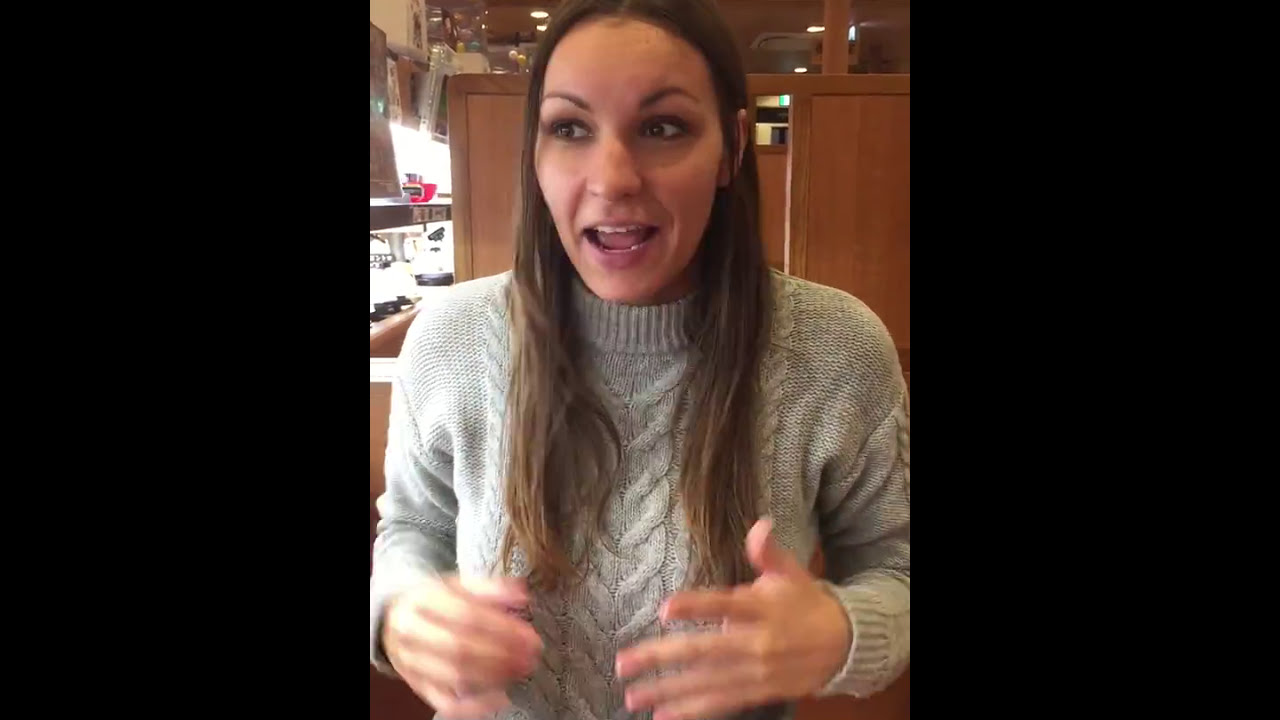The image captures a dynamic moment of a Caucasian woman, appearing to be between 25 and 40 years old, with long brown hair cascading over her shoulders. Her expressive face, marked by brown eyes and open mouth, suggests she has just been surprised or is in mid-conversation. She is adorned in a gray, knitted sweater, and her hands are blurred, indicating she's gesturing energetically. She seems to be looking slightly to the right, engrossed in an animated dialogue.

The background features elements that hint at an indoor setting, possibly a store or a kitchen. Behind her, there are light brown wooden cabinets or partitions and assorted trinkets, possibly hinting at a restaurant setting due to a visible buffet area to the far left. The lighting in the image appears to stem from above, casting a soft glow on her expressive posture. The overall effect is that of a snapshot taken in the middle of an engaging moment, capturing both her animated expression and lively hand motions.